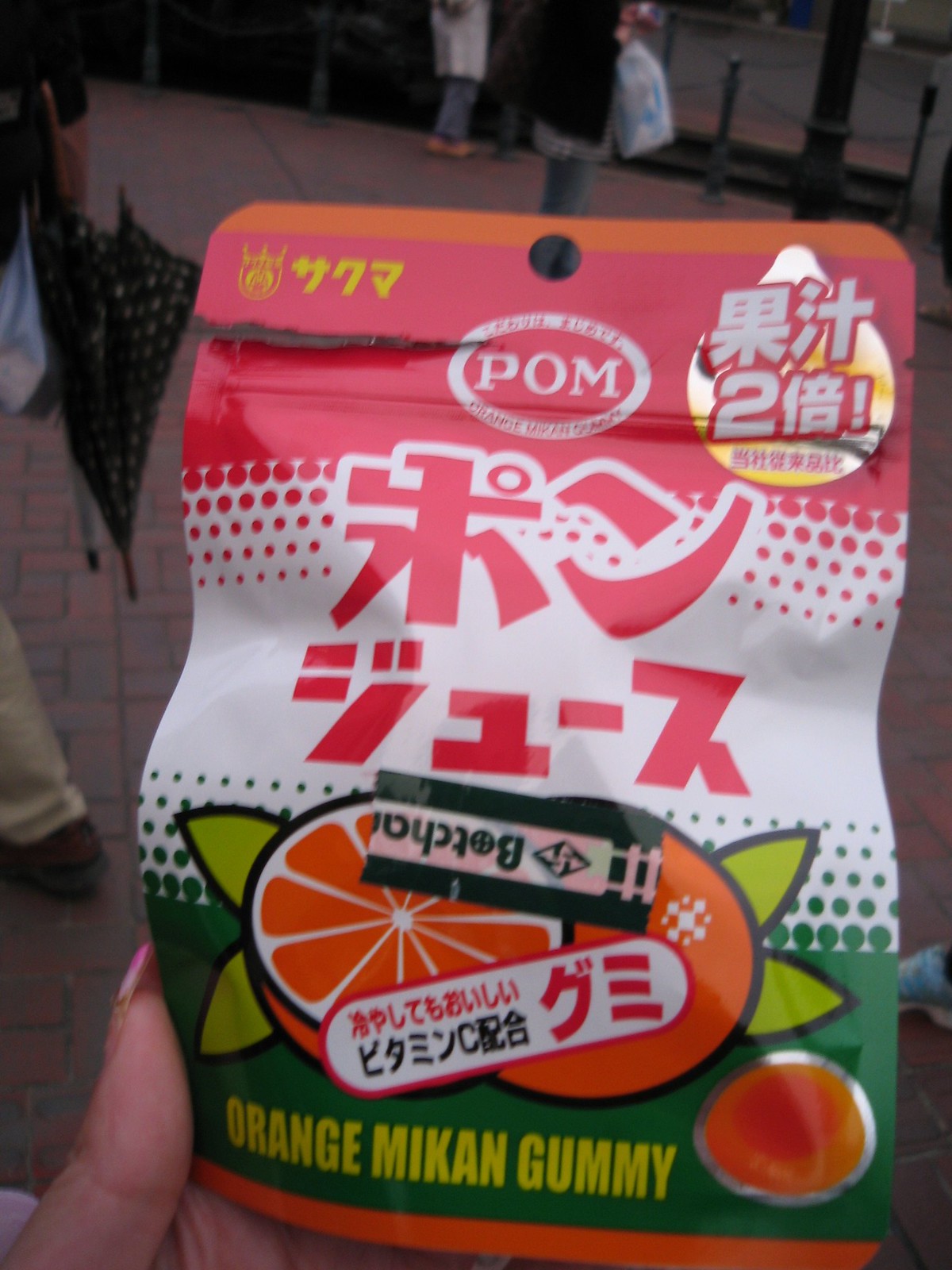This photograph captures a person holding an opened bag of Orange Mikan Gummy candy. The bag, which is pink, orange, and white, is adorned with detailed Asian characters in red on a white background. At the top of the bag, "POM" is written in white letters within a red circle, and above it, the number "2!" is visible. The top left corner features yellow characters, while the top right corner has white characters outlined in red. The candy bag showcases an image of an orange, outlined in black with two green leaves behind each half, positioned on a green banner at the bottom that contains the product name in yellow writing. Nearby, there's a circular silver emblem showing the gummy candy itself. The package is held in the person's palm, with their thumb and long decorative fingernail clearly visible. In the background, you can see a brick surface and a person walking with a tan pair of pants and a brown shoe, holding an umbrella on her back. The image is detailed, revealing even the tiny red and green dots at the top and bottom parts of the bag.